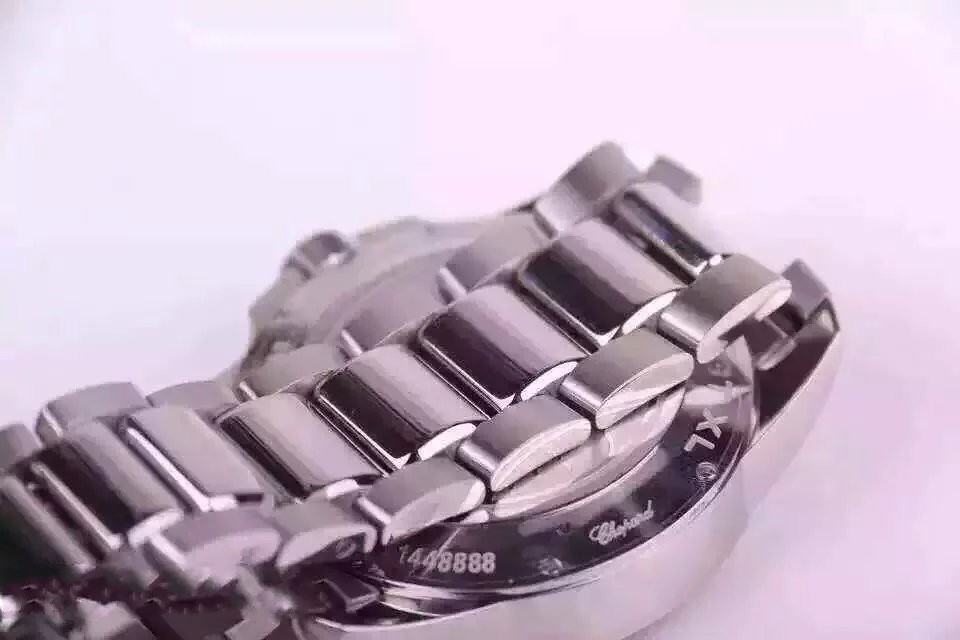This close-up photographic image features an analog watch resting on a white surface with a matching white background. The watch is flipped upside down, displaying its silver-toned, chrome-finished back and metal band. The band is composed of three types of links: larger, horizontally aligned central links flanked by smaller, vertically aligned side links, giving it a distinctive chain-like appearance. Detailed writings and etchings are visible on the watch back, including the numbers "1448886" near the bottom center and "XL" along the top right. Although some text appears to be the designer's name, it remains partially unreadable but might resemble "Clifford." A reflective silver knob is noticeable on the top left part of the watch. The overall construction and aesthetic underscore its sophisticated metal craftsmanship.